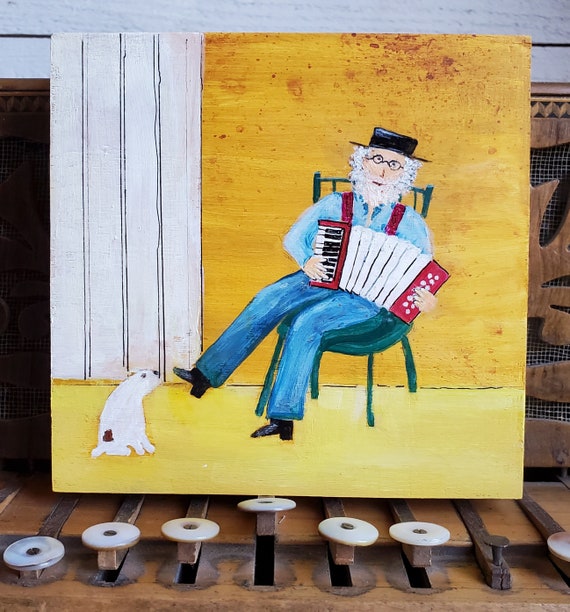This photograph captures a quaint artwork resting atop an old accordion. The small painting, seemingly on a wooden square canvas, depicts an elderly man with a white beard and mustache, donning a black hat, black thin-rimmed glasses, blue jeans, black pointed boots, a light blue shirt, and red suspenders. He is seated on a bluish-green chair, playing an accordion. His right hand is positioned on the keyboard while his left hand manages the keys of this predominantly white accordion, accentuated by red trim around the keyboard and back keys. A small white dog with a black spot above its tail sits attentively at the man's feet, gazing up at him.

This miniature scene is set against a simple backdrop featuring four vertical white wooden planks to the left, meeting a yellow wall that extends to a yellow floor. The painting rests against an intricately detailed accordion characterized by its wooden structure and ivory or plastic buttons, one of which is missing. The elements of the photograph combine seamlessly to highlight the rural, folksy charm of the depicted scene.